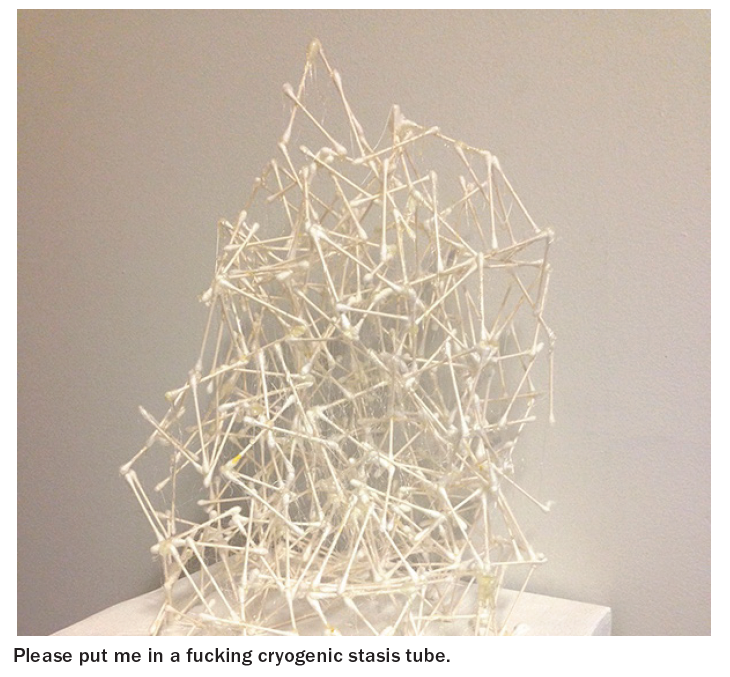The square image presents a curious white sculpture, seemingly constructed from an estimated 200 Q-tips, arranged in a chaotic, vertically rising structure. The sculpture, approximately a foot high, stands on a white table or flat surface, which serves as its base. The background is a dark gray to beige-gray, creating a stark contrast that highlights the predominantly white assembly. The Q-tips are inserted in a seemingly random yet intricate manner, losing symmetry as they ascend from the bottom, where a hint of a circular base can be seen. Across the bottom of the photograph, in bold black print, are the cryptic words: "Please put me in a fucking cryogenic stasis tube.", adding a layer of enigmatic context to the composition.